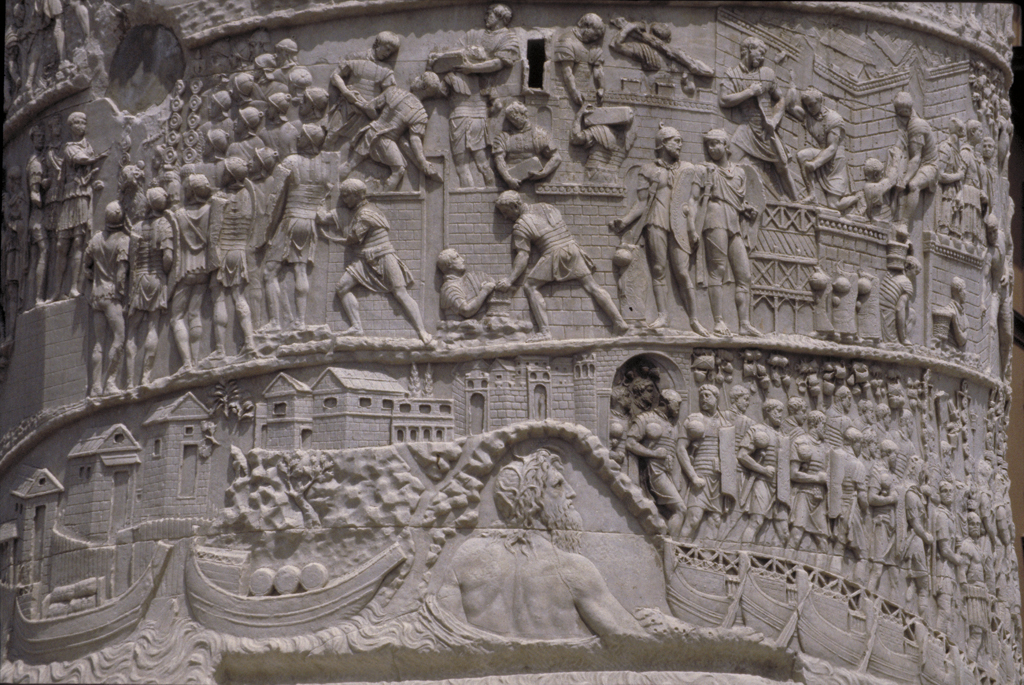This image showcases the intricately carved Trajan's Column, an iconic monument from the early Roman Empire. The column stands as a single, towering entity, adorned with detailed relief carvings that spiral around its marble or stone surface. The background exhibits a consistent stucco beige-brown hue. The carvings are organized into two primary scenes: 

The top portion depicts various Roman soldiers in differing attire, some bearing helmets and weapons, engaging in combat or standing in line as if prepared for battle. A prominent figure, shown from behind, displays his right profile with a bearded face and wavy hair, possibly representing a deity or significant historical figure, overseeing the scene from what appears to be a parapet.

The bottom section features a series of small houses lining the left side, indicative of domestic life or structures during that period. On the right side, palace guards are depicted exiting a grand structure. At the very base, houses blend into a waterfront scene where boats are present. A notable figure, who may represent a god such as Neptune or Zeus, emerges from the water—his upper back and head turned away from the viewer, contributing to the grandeur and depth of the depicted narrative.